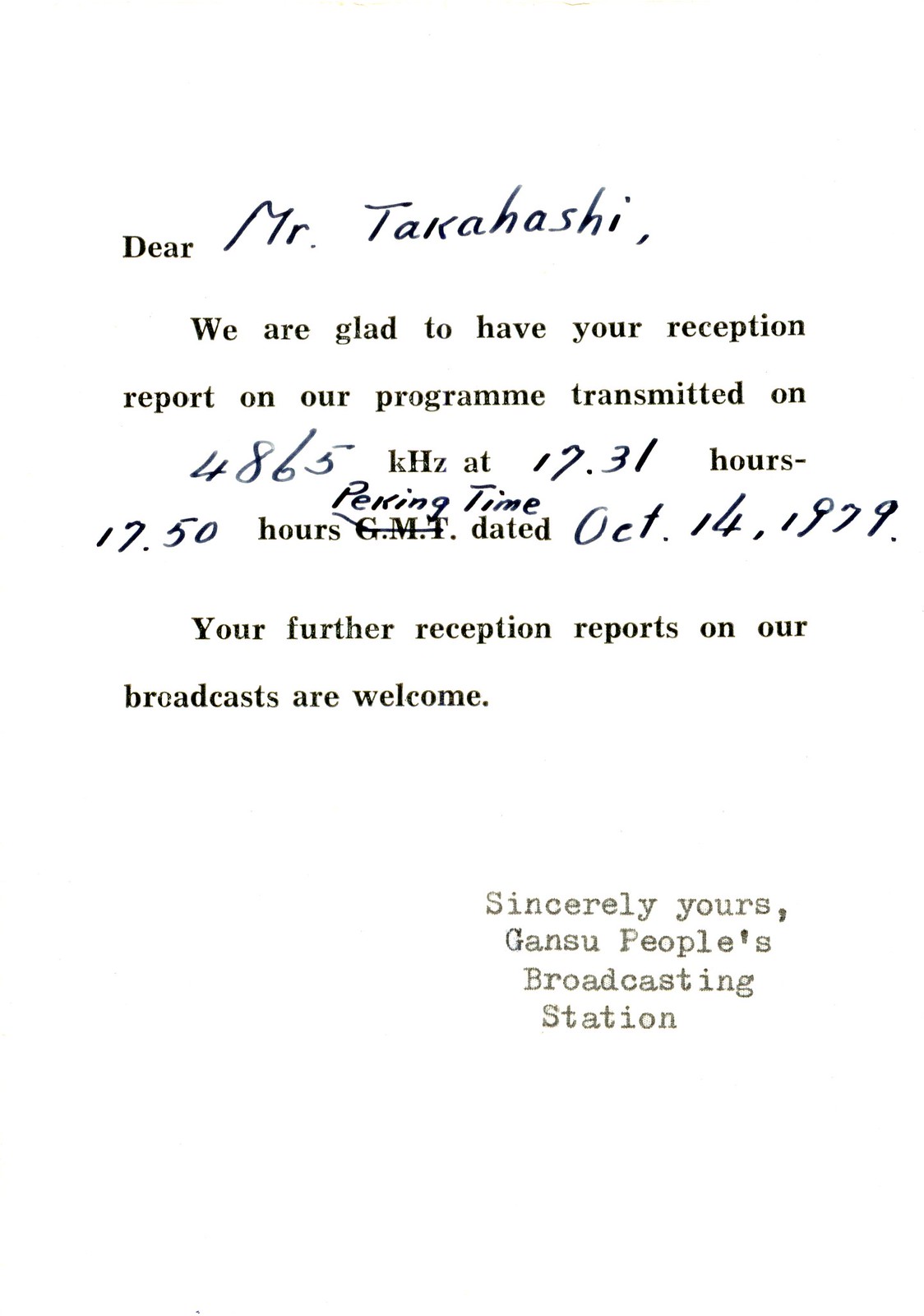The image depicts a formal letter from the Gansu People's Broadcasting Station, addressed to Mr. Takahashi. The text is presented in black ink on a white background, with certain sections handwritten, suggesting modifications made post-typing. The letter expresses appreciation for Mr. Takahashi's reception report of a broadcast transmitted on 4,865 kilohertz at 17:31 hours to 17:50 hours, Peking time, on October 14, 1979. The letter welcomes further reception reports from Mr. Takahashi. Notably, the greeting "Dear Mr. Takahashi" is partially handwritten alongside the typed text. Additionally, the notation of Peking time is manually corrected over an initial GMT label. The letter concludes with "Sincerely yours," followed by a typed signature from the Gansu People's Broadcasting Station.